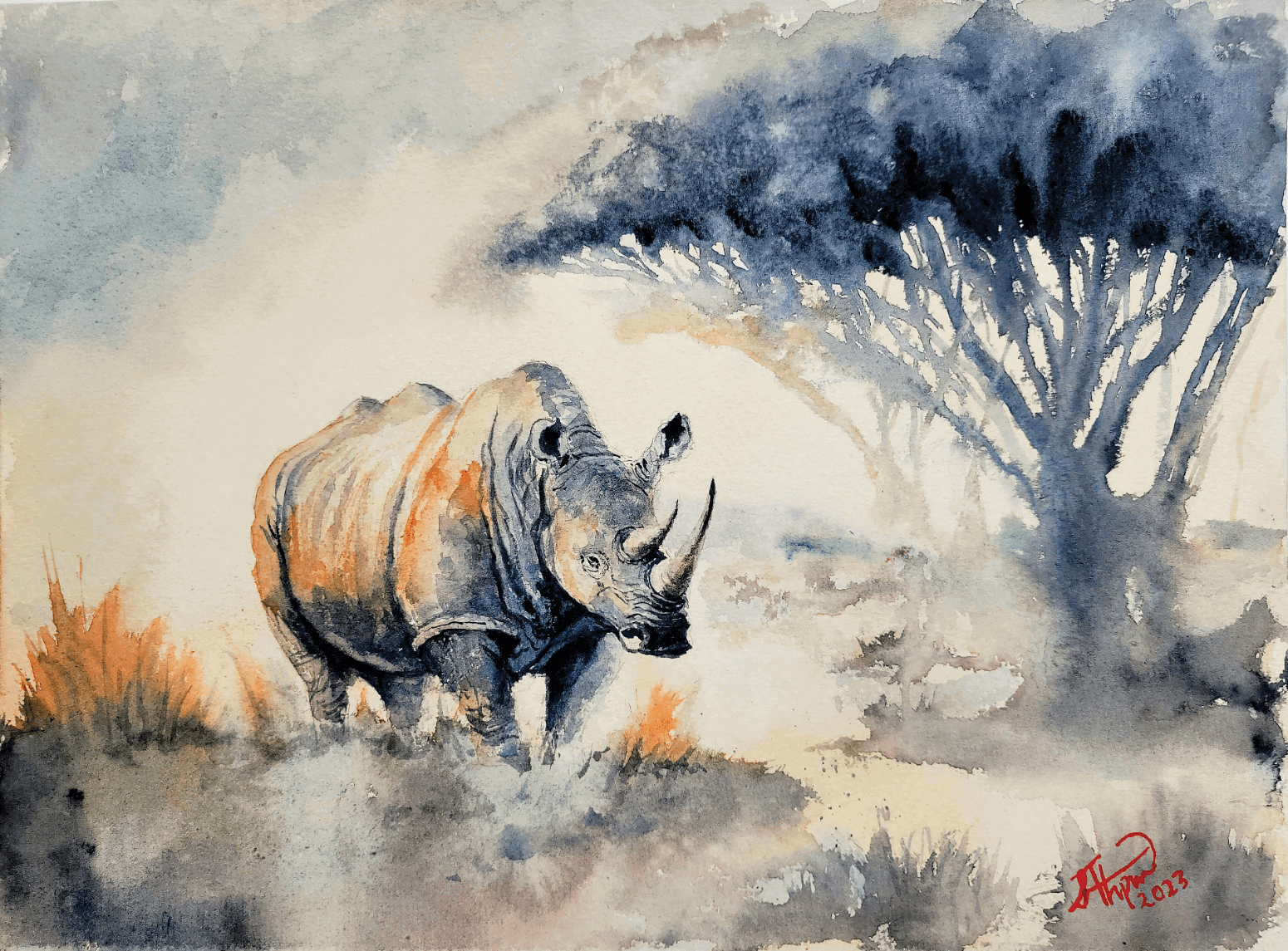This painting portrays a rhinoceros traversing the plains, likely evoking the landscapes of Africa. The rhino, positioned on the left side, strides toward the right, with its sturdy form detailed in shades of gray and white, accentuated by vivid orange highlights. These orange tones are replicated in the shrubs and weeds around it, suggesting the warm glow of morning light. The rhino’s two horns, prominent ears, and textured hide are meticulously rendered, contrasting with the rest of the scene's more abstract, watercolor-like quality. The ground and sky, both awash with swirling gray and white hues, blend seamlessly, making it challenging to distinguish between them. To the right of the rhino stands a dark tree, fading into the background amidst lighter, almost ghostly trees, alluding to an African savanna. In the bottom right corner, the artist's signature and the date '2023' are inscribed, confirming its recent creation.